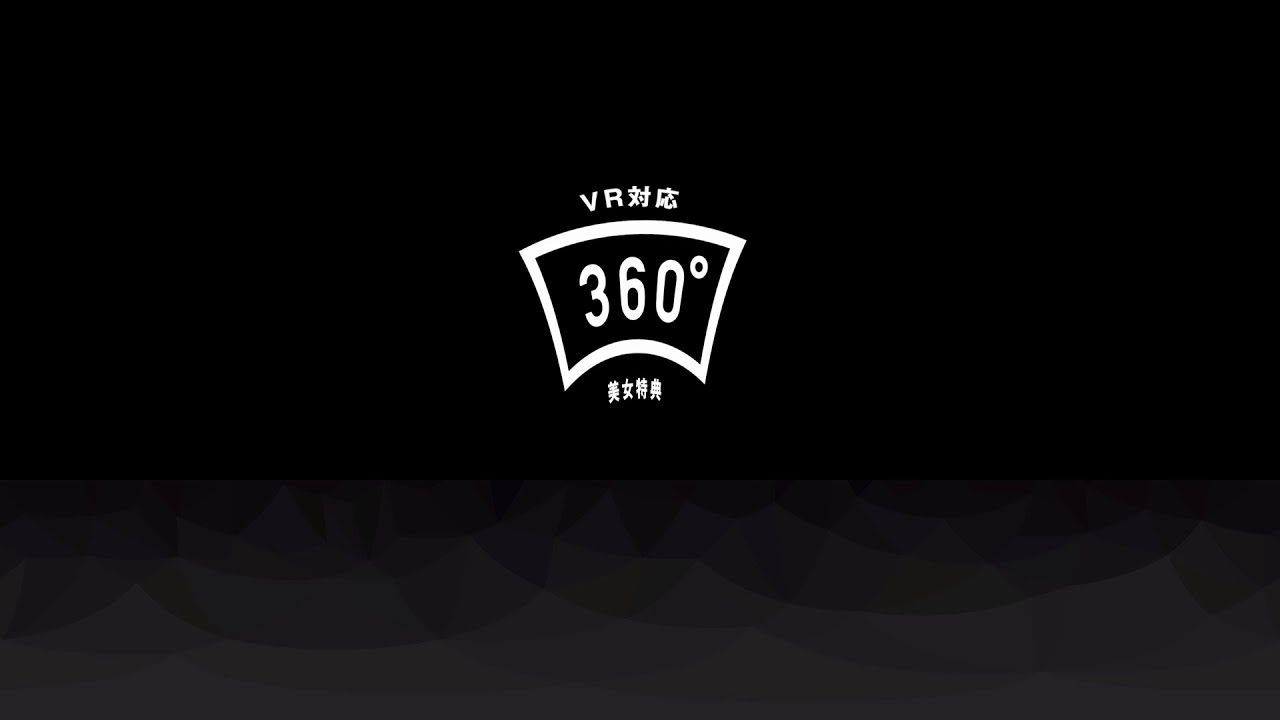The image is a screenshot of a digital logo set against a black background that gradually fades to gray toward the bottom. At the center of this image, there is a white rectangular shape approximately one inch by one inch. Inside the rectangle, the text "360°" appears prominently in white, denoting 360 degrees without specifying a measurement unit such as Fahrenheit or Celsius. Above the number, the letters "V" and "R" are positioned. Flanking these elements is text in an oriental language, likely Chinese, with two characters at the top and four characters below the number "360°." The white text is neatly enclosed within the white rectangular border, and no other objects or text are present in the image. The aesthetic of this logo suggests it could belong to a company, possibly related to virtual reality. The overall design and composition of the image lend a crisp, digital appearance, resembling clipart or a stock image asset.